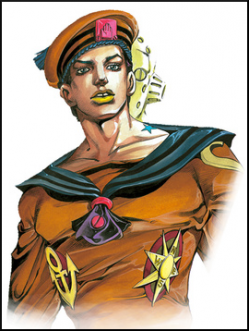This image features an animated or cartoon drawing of a muscular white man with light skin, wearing a brown jersey adorned with a gold anchor and a gold star on his midsection. His lips are notably bright yellow. He is dressed in a tight orange shirt and has a dark teal scarf elegantly draped around his shoulders, tied in the front with a pink tie, tapering into a purple and black section below. The man is wearing a brown hat reminiscent of a beret or old sailor cap, distinguished by a pink emblem in front, surrounded by a dark teal band above his forehead. The background is white with a black border, thicker on the sides. Peeking over his shoulder is a yellow cat-like eye, suggestive of a robot's head, adding an intriguing layer to the image.